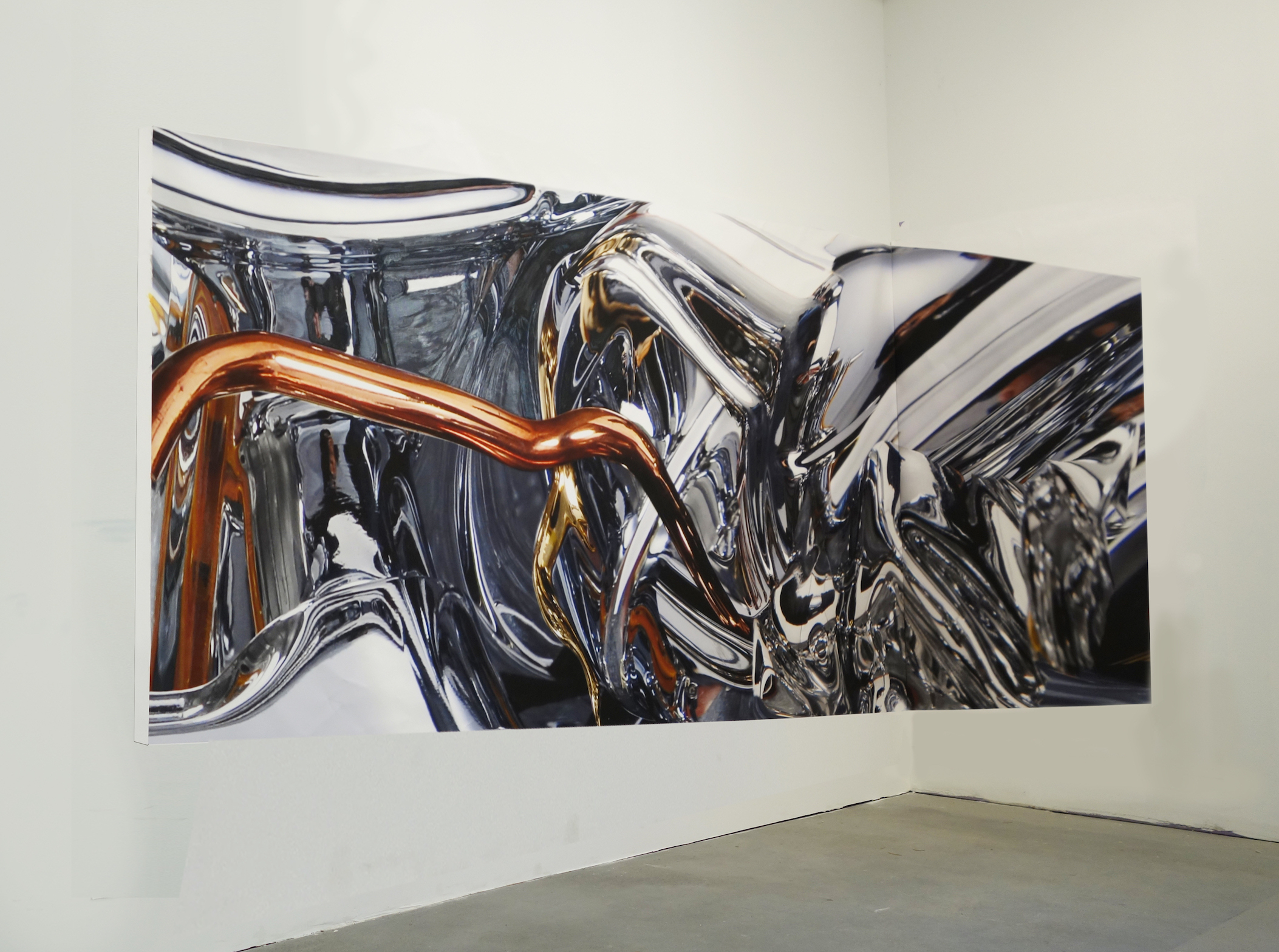This image showcases an abstract art piece in an art gallery with an exposed concrete floor and pristine white walls. The artwork intriguingly spans across a corner, with about 75% of it on the left wall and 25% curving onto the right, creating an engaging visual seam where the two walls meet. The large, horizontally oriented canvas depicts a mesmerizing array of shiny, metallic tubes in vibrant shades of orange, bronze, gold, and silver, giving the impression of being copper, chrome, and gold. These reflective tubes appear to twist, turn, and jumble together in a complex, visually stimulating pattern that evolves and becomes increasingly distorted towards the right side. The background seems to feature a gray, distorted texture, enhancing the piece's abstract nature. The overall effect is one of a dynamic, trippy, and highly reflective metallic landscape, seamlessly integrated into the gallery's modern space.